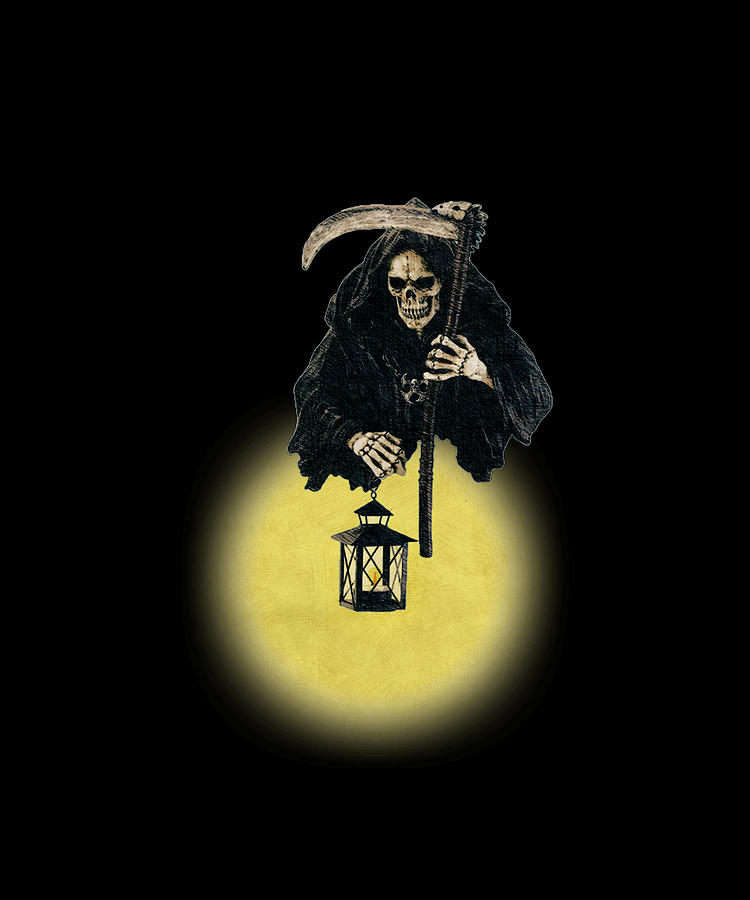This digital image depicts the Grim Reaper in vivid detail against a pitch-black background. Centered in the composition, the Grim Reaper is shown from the waist up, clad in a traditional hooded cloak that conceals much of his skeletal form, revealing only his skull face and bony hands. His expression seems to be one of a grim smile as he looks down at a lantern held in his right hand. This lantern emits a circular glow of yellow light, which contrasts strikingly with the dark surroundings. The lantern itself features intricate black metal detailing and holds a candle at its heart. In the Grim Reaper's left hand is a staff with a long bone crook, possibly a scythe with a blade seemingly made of bone and a handle resembling finely detailed black wood. The yellow light emanating from the lantern bathes part of his form, highlighting the eerie and haunting aura of this skeletal figure.